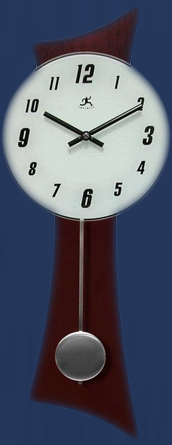This long, rectangular vertical photograph showcases a mid-century modern wall clock set against a dark blue background. The wooden clock features a curved, angled base and top that slopes downwards at the bottom and upwards at the top. Dominating the design is a large, slightly oval, white clock face near the top, marked with black numbers around its edges. The black clock hands indicate the time as 10:10. Below the "12" on the clock face, there is a black figure of a person running to the right, with their left arm bent down and right arm bent up. Extending from the bottom of the clock face is a thin silver bar that culminates in a round silver disc, forming the pendulum. The overall shape of the clock includes a dark brown, curved rectangular body.